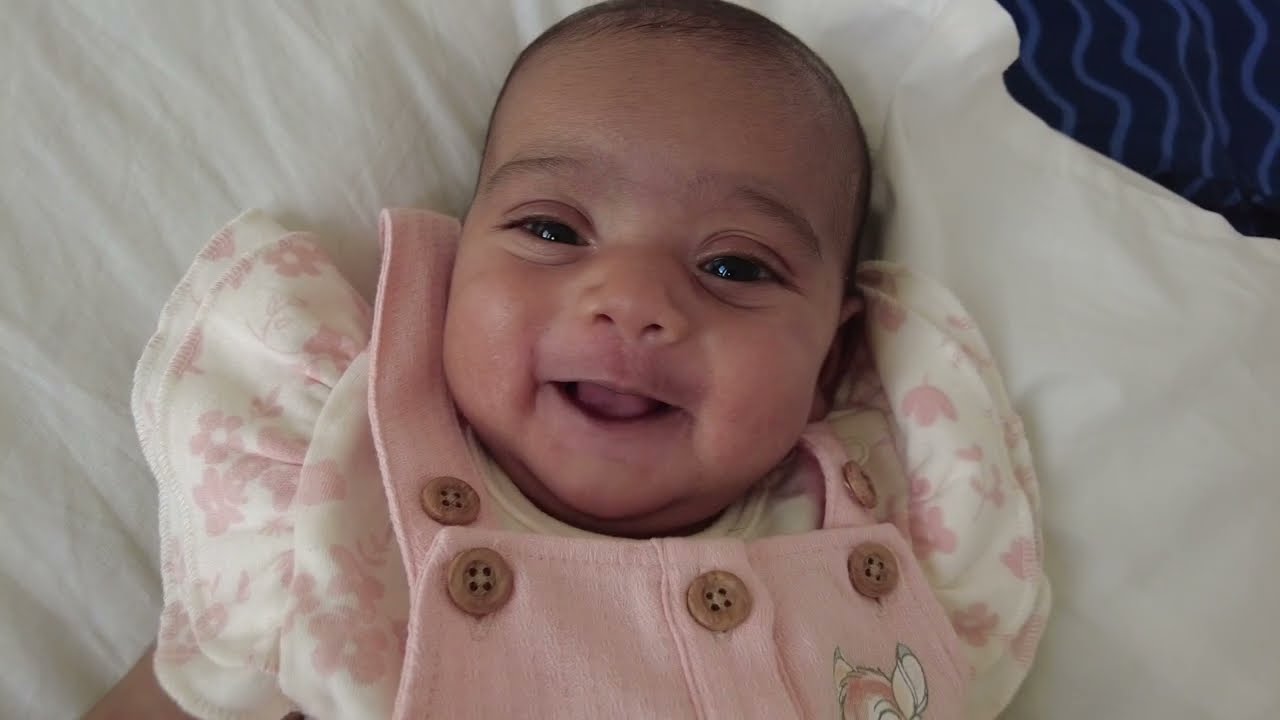The image features a close-up view of an infant girl, laying on her back with a joyful smile. Her dark hair and big dark eyes are complemented by her long eyelashes, and her little tongue is visible. She is dressed in a pink outfit with frills around the shoulders, adorned with a darker pink floral design. The outfit includes a pink bib-style jumper secured with five tan buttons, arranged on the shoulder straps. On the left side of her bib, there is a partially visible cartoon character resembling a deer or chipmunk with white ears and brown fur. The baby rests on a white sheet or comforter, with a dark blue fabric featuring light blue wavy lines located in the top right corner of the image. The photograph captures her from chest up, centered on her beaming face, and it's evident that the photographer is positioned directly above her.